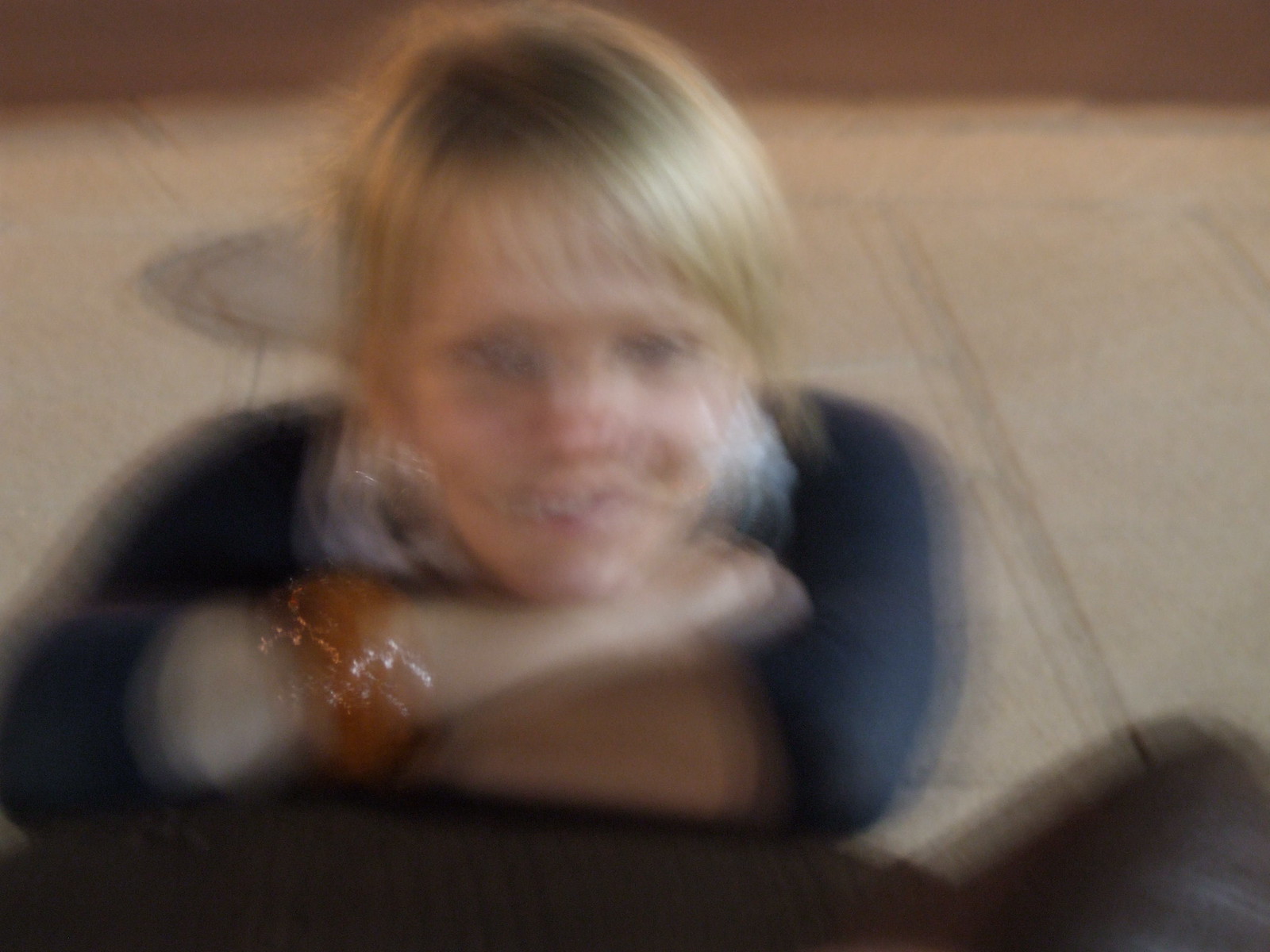This is a color photograph featuring a close-up of a young girl, likely around 12 years old. Despite the image being very blurry and out of focus, some details are discernible. The girl is caucasian with short, blonde hair cut in bangs, and her hair length does not extend below her ears. She is wearing a dark blue shirt that reaches just below her elbows. Her arms are folded in front of her, and she is resting her chin on her cradled arms. On her right wrist, she is wearing a bracelet that seems to be gold in color. The background, although indistinct, appears to show a light brown, hardwood floor.